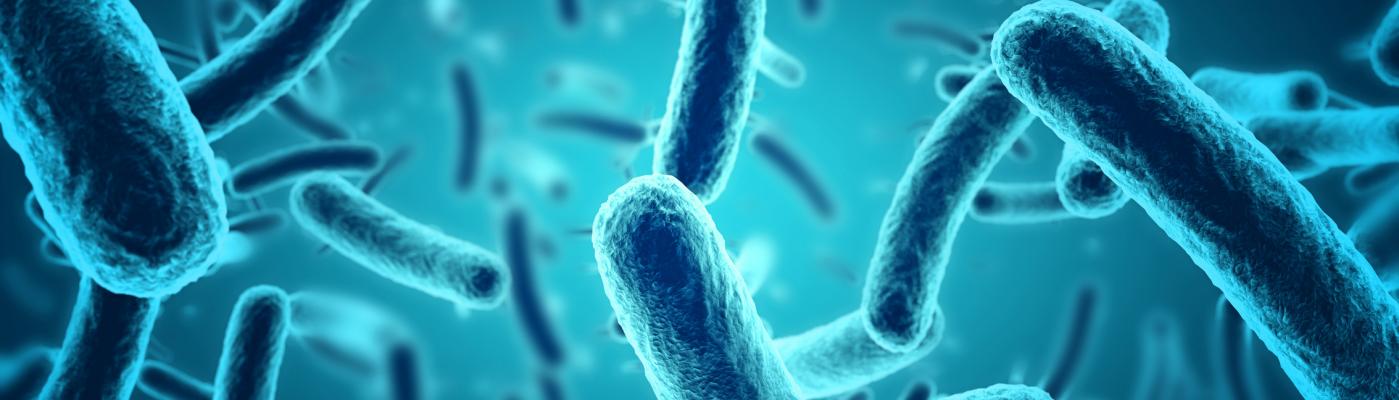This digitized close-up image, reminiscent of a microscopic view, showcases numerous blue elongated ovals that resemble puffed Cheetos or hot dogs. The main color palette is blue, ranging from deep, almost black, hues to lighter sky blue shades, with some ovals even having a white outline. The ovals vary in orientation, with some prominently protruding and extending across the image, such as the one starting from the center-right and descending to the lower right corner, and another from the upper left extending downwards. The texture of these shapes is noticeable, adorned with line-like markings. The background is lighter blue, and the clarity of these shapes diminishes as they fade into the background, creating a sense of depth. This detailed view brings to life the mysterious, intricate world visible under a microscope.